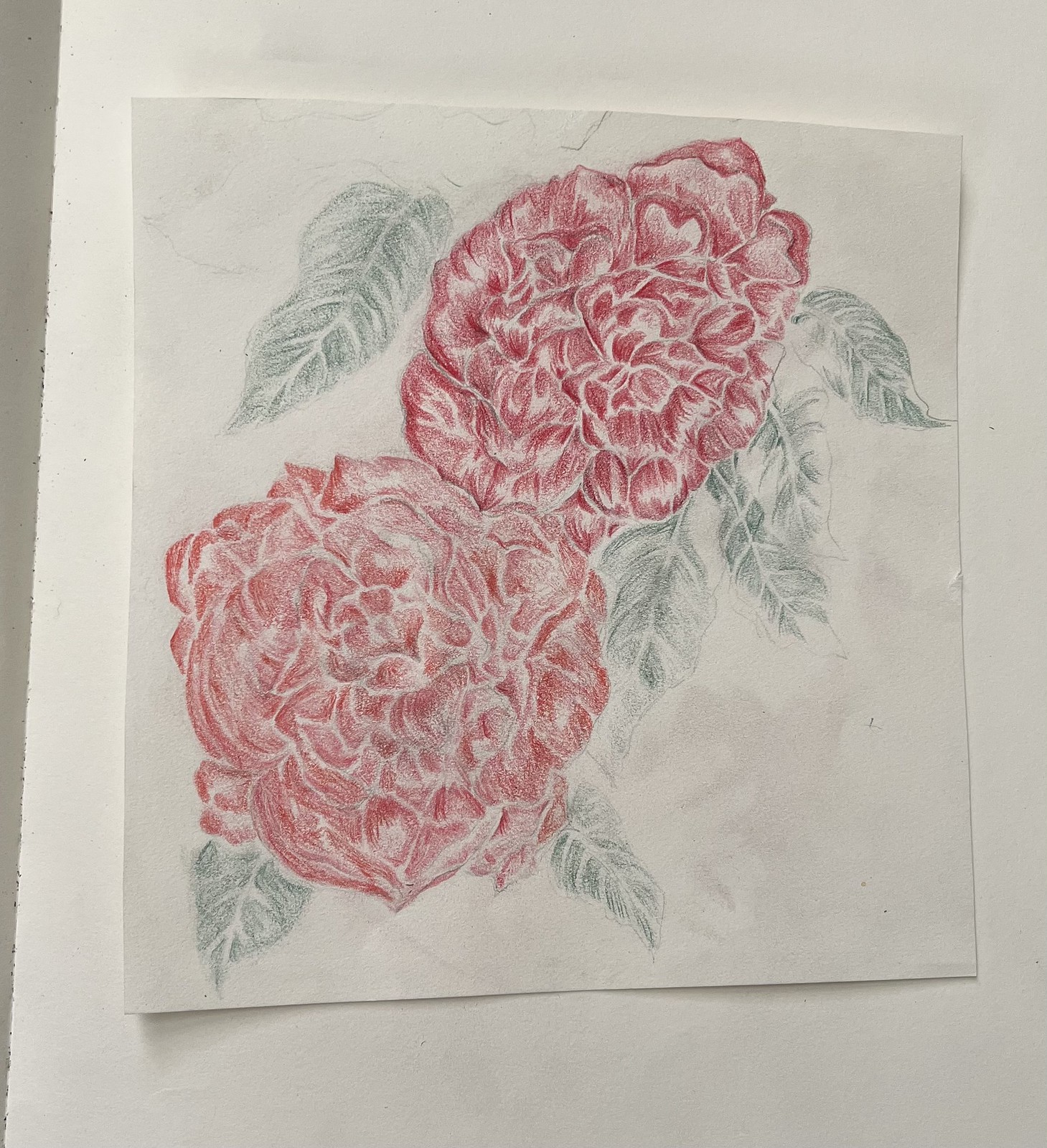The image is a close-up indoor photograph taken during the daytime of a detailed and professional-looking drawing or painting lying flat on a white table. The artwork features two large red flowers, resembling either carnations or peonies, intricately colored with red and white highlights that accentuate the individual petals. The flowers are surrounded by several green leaves, which have been meticulously shaded with both dark green and white to illustrate the veins and add depth. The background of the paper is white, with some hand smudges noticeable around the leaves, and a touch of gray is visible on the left side of the table. The composition is square with a white paper base, providing a clear and clean background for the vibrant floral depiction.